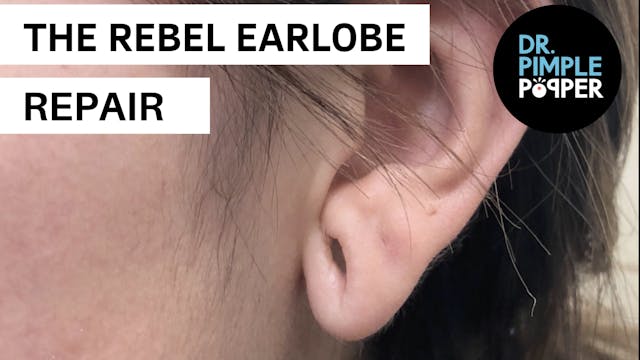The image is a close-up photograph of someone's left ear with pale skin and brown hair that features stray strands from their sideburns. In the upper left corner, there are two white banners with black, all-capital letters. The top banner reads "THE REBEL EARLOBE" and the bottom banner reads "REPAIR." The photo highlights the earlobe, revealing two small piercings on the upper part and a significantly larger hole, roughly finger-width, at the bottom, indicative of past use of large gauge earrings. In the upper right corner, there's a black circle with the logo and text "Dr. Pimple Popper," where "Dr. Pimple" is in blue and "Popper" is in white, serving as an advertisement for the TV show.